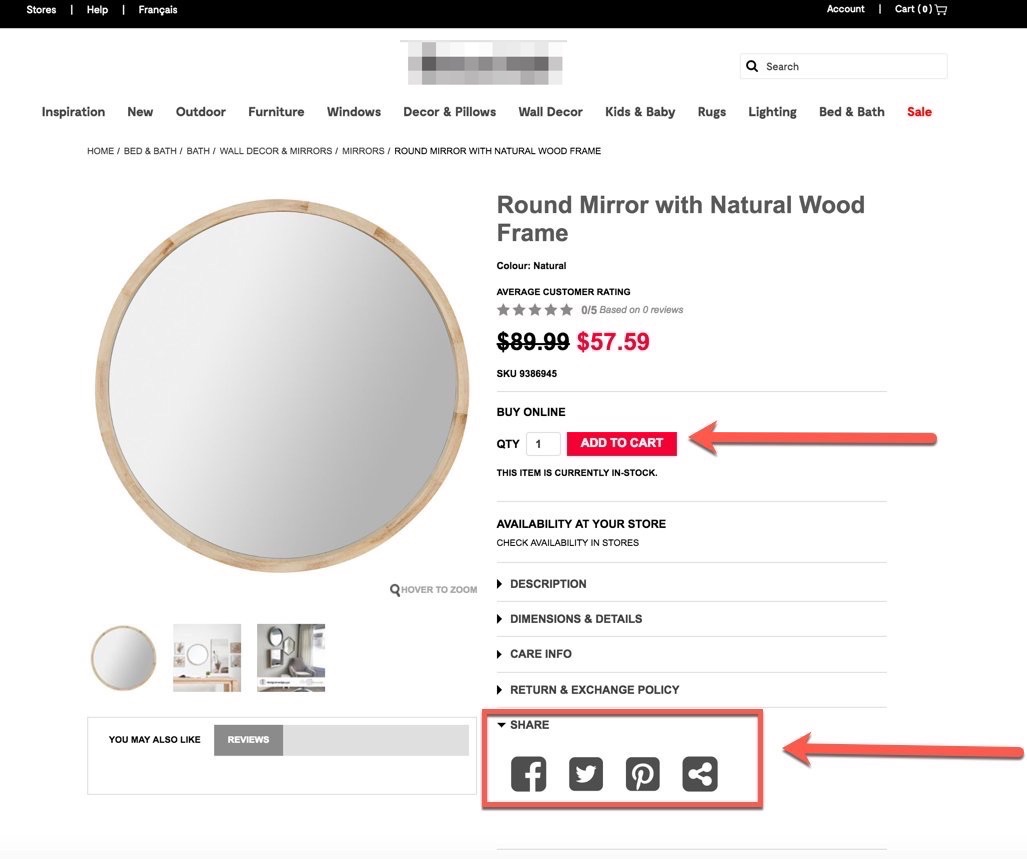This is a screenshot of a product page from a website. The top portion features a black bar spanning the width of the page. On the top left of the bar, there are three clickable options labeled "Stores," "Help," and "Front Saw," all in white text. The top right of the bar shows two buttons: "Account" and "Cart," also in white.

In the center of the top section, the website's name is obscured. Beneath the black bar, the rest of the page is primarily white. The white section begins with a prominent search bar located on the top left. Directly below the search bar is a horizontal navigation menu featuring black buttons with white text. The buttons are labeled "Inspiration," "New," "Outdoor," "Furniture," "Windows," "Decor," "Pillows," "Wall Decor," "Kids & Baby," "Rugs," "Lighting," "Bed & Bath," and an additional button labeled "Sale," which is highlighted in red.

Further down the page, the main product image appears—a round mirror with a wooden frame displayed on the left side of the screenshot. Accompanying the image, to the right, is a description stating "Round Mirror with Natural Wood Frame."